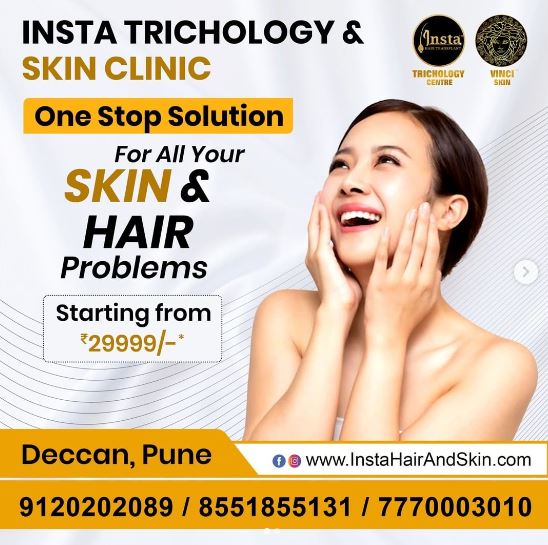This image is a promotional advertisement for Insta Trichology and Skin Clinic, designed with a silky, creamy-white background reminiscent of luxurious fabric. Dominating the top of the graphic, text in various fonts and sizes reads, "Instant Trichology and Skin Clinic - One Stop Solution for all your skin and hair problems." Below this, it mentions services starting from 29,999 (with an unrecognized currency symbol). 

On the right-hand side, a vibrant photograph captures a young, smiling Asian woman with glowing skin, her hands gracefully touching her face as she gazes upwards. Overlaying the image are round symbols, possibly indicating "Trichology Center" and "Vinci Scion." 

Towards the bottom, a yellow-orange banner features the text "Deccan, Pune" followed by three sets of long phone numbers separated by slashes: 912-020-2089 / 855-1855-131 / 777-000-3010. The URL for more information, www.instahairandskin.com, is prominently displayed beneath the contact numbers.